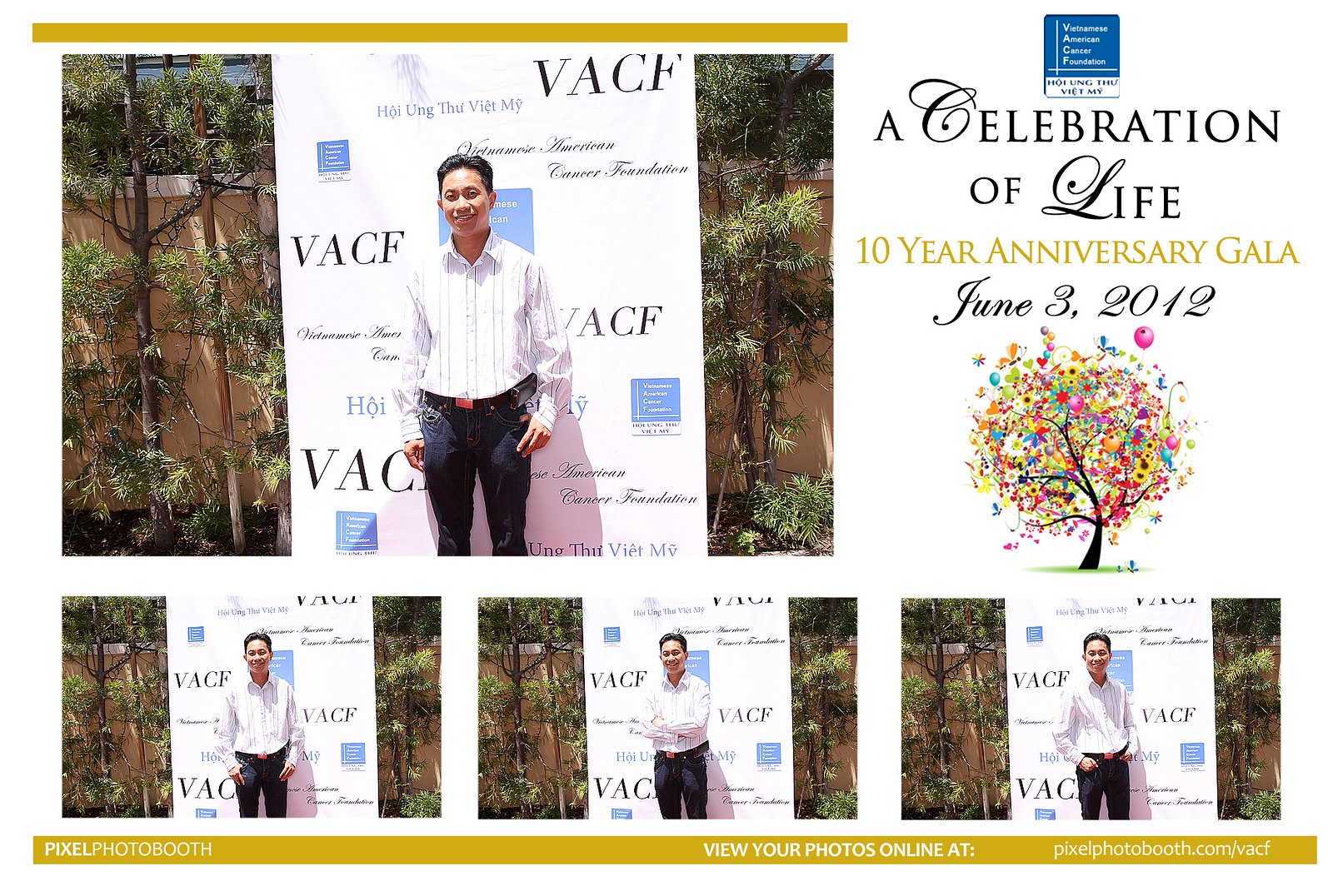The image is a photo booth promotional card for the Vietnamese American Cancer Foundation (VACF) 10-Year Anniversary Gala held on June 3, 2012. The card features a thin golden border framing the top and bottom. On the upper left side, there is a large photograph of an Asian man with short black hair, parted to the side, wearing a light-colored button-down striped shirt and dark pants. He stands in front of a hanging banner decorated with the VACF logo and initials, positioned before a short wall with trees behind it. 

To the right of the large photograph, the card’s upper section contains text in black and gold fonts reading "A Celebration of Life, 10-Year Anniversary Gala," followed by the date, June 3, 2012. Below the text, there is an artistic depiction of a tree with a black trunk and branches, adorned with multicolored leaves in pinks, yellows, greens, and blues.

The bottom section of the card features three smaller, identical photographs of the man in various poses, standing in front of the same banner. The bottom golden border includes additional information in white text about the photo booth, instructions to view photos online, and a website address. The overall design emphasizes the celebratory and commemorative nature of the event while promoting the Vietnamese American Cancer Foundation.